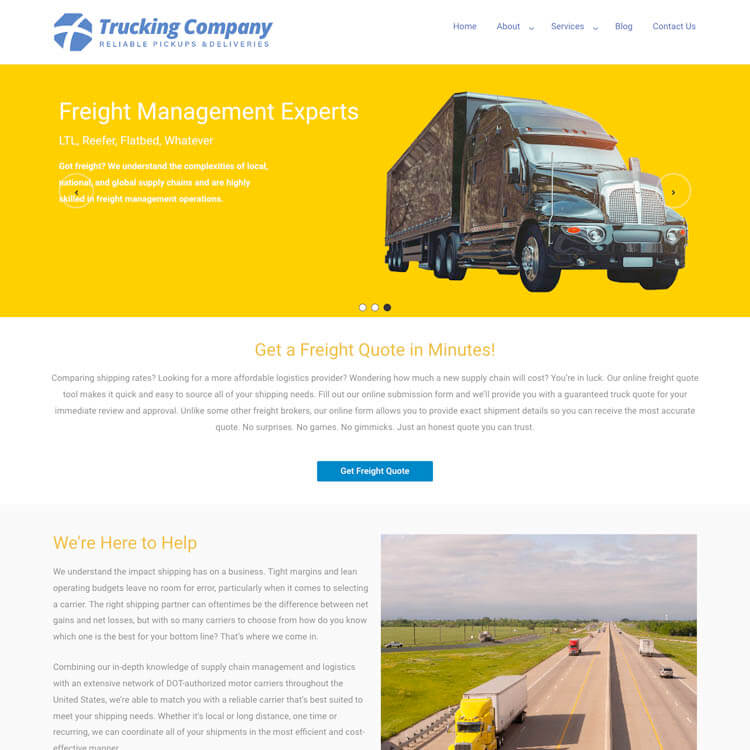Screenshot of a Trucker Express Website Homepage:

This screenshot captures the homepage of a trucking company’s website, dynamically designed with a professional yet straightforward aesthetic. The central element is a bold blue logo set against a clean white background, flanked by a minimalist top navigation menu. The menu includes options labeled "Home," "About," "Services," "Blog," and "Contact Us," with dropdown indicators next to "About" and "Services" for further subcategories.

Dominating the visual space is a striking header image featuring a sleek black commercial freight truck set against an eye-catching, vibrant yellow background. Overlaid on this image is white, bold text proclaiming "Freight Management Experts." Directly beneath this header, there is additional text intended to provide further details, but it is unfortunately marred by heavy JPEG artifacts, rendering it unreadable.

Below the main header, a standout section invites potential clients to "Get a Freight Quote in a Minute." This section comprises a succinct gray descriptive paragraph and a central blue call-to-action button with white text that reads "Get Freight Quotes." 

Proceeding down the page, a section with a gray background features the prominent yellow header "We're Here to Help," which introduces another detailed paragraph of helpful information. Beside this text block, to the right, is an evocative photo depicting trucks cruising down a sun-drenched highway, reinforcing the theme of efficient and reliable freight transportation.